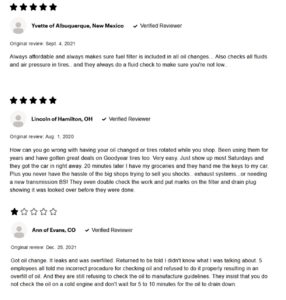**Caption: A Tale of Two Reviewers – Yvette from Albuquerque vs. Anne from Evans, Colorado**

Yvette, a verified reviewer from Albuquerque, has consistently praised her local auto maintenance shop for their exceptional service. Yvette highlights their comprehensive oil change service, which not only includes the replacement of oil and fuel filters but also thorough checks of all fluid levels and tire air pressure. Yvette appreciates the convenience of getting her car serviced while shopping, noting that the entire process, including tire rotations and oil changes, typically takes around twenty minutes – just enough time for her to complete her grocery run. She has experienced no high-pressure upselling tactics and values the double-checking process, where marks are placed on the oil filter and drain plug to indicate thorough inspection. Yvette’s repeated patronage, spanning several years and including purchases of high-quality Goodyear tires, underscores her satisfaction and earns the shop a five-star rating from her.

In contrast, Anne, another verified reviewer from Evans, Colorado, recounts a distressing experience with the same shop. Anne’s visit resulted in an oil leak post-service, and she felt patronized and dismissed by the staff when she raised her concerns. The employees allegedly refused to follow proper oil-checking procedures, contradicting manufacturer guidelines by not waiting the recommended five to ten minutes for the oil to settle. This unfortunate encounter left Anne "petrified" and dissatisfied, leading her to give the shop a one-star review. 

Their experiences highlight the contrasting service perceptions, demonstrating that customer service can vary greatly even within the same establishment.